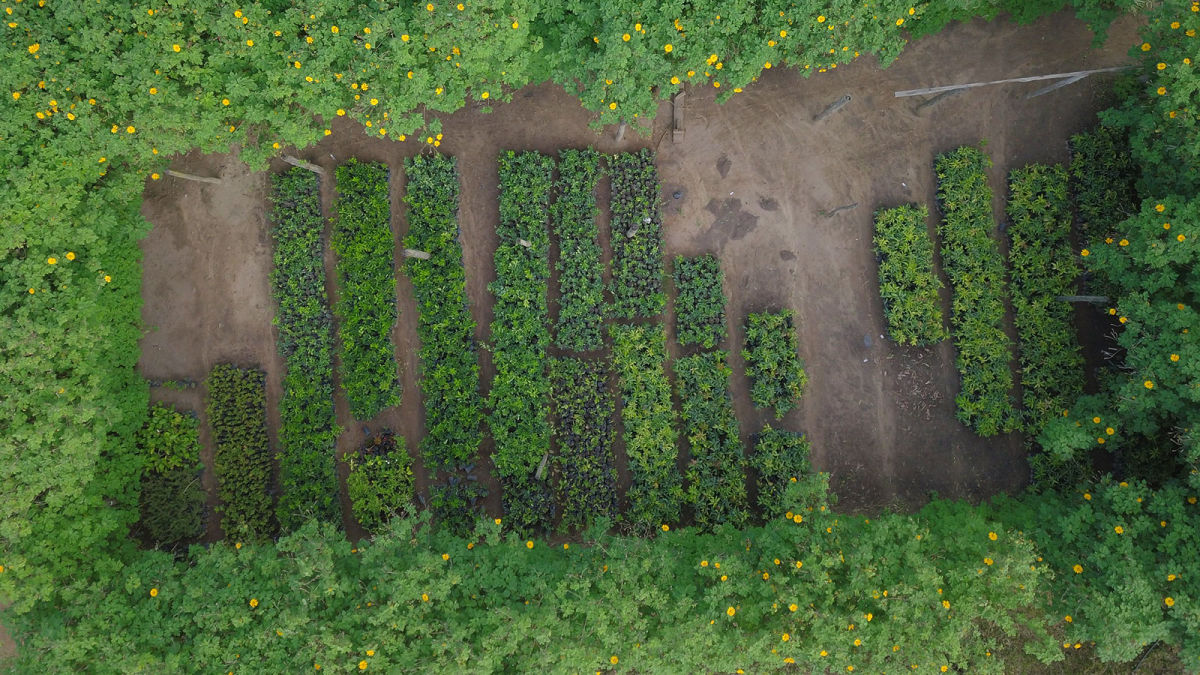This overhead photograph captures a lush garden, possibly a nursery, surrounded by dense green shrubbery adorned with small, delicate yellow flowers. In the center of the image, a dirt patch features several rectangular garden beds filled with similar green bushy plants. A notable aspect in the top right corner shows a pathway leading to a broad, gray surface, which could be a concrete or asphalt patio. This patio area contains multiple rows of plants arranged in various lengths—some stretching nearly the full width of the space, suggesting they might be adjustable or movable storage units for plants. Amidst this organized chaos, there appears to be a large, metallic, stencil-like structure adding an intricate yet unclear element to the scene.